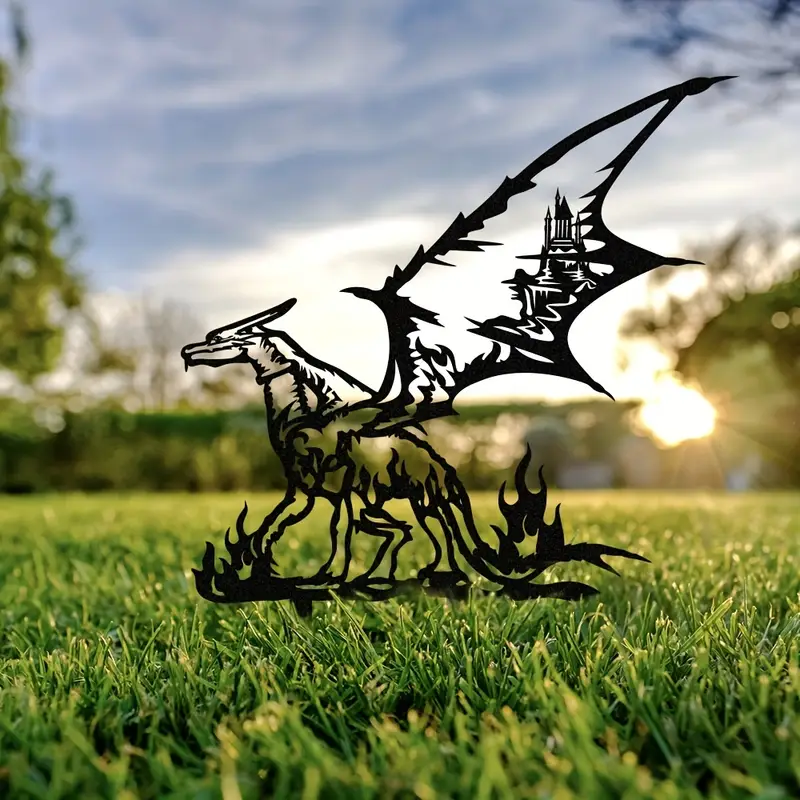This captivating photograph features a detailed, two-dimensional metal dragon sculpture placed in a lush, high-quality grassy field. The grass is so sharply focused that you can almost count individual blades, offering a stark contrast to the blurred background, where vague shapes of trees and hedges are barely discernible. The sky, a grayish-blue, has the sun peeking through in the bottom right corner, casting a bright, amorphous glow.

The dragon, facing left, is meticulously crafted, appearing hollow and black, which allows the viewer to see through to the other side. Its posture suggests it's sitting, making it resemble yard art. The dragon's design includes intricate cutouts, with flames adorning its feet, tail, and front right paw, and a striking silhouette of a castle nestled within its single visible wing. The castle appears to be perched on a mountain, complete with waterfalls cascading down, adding to the fantastical element of the piece. The dragon's elongated, lizard-like face and the spikes emerging from its base further enhance the mystical and artistic allure of the sculpture.